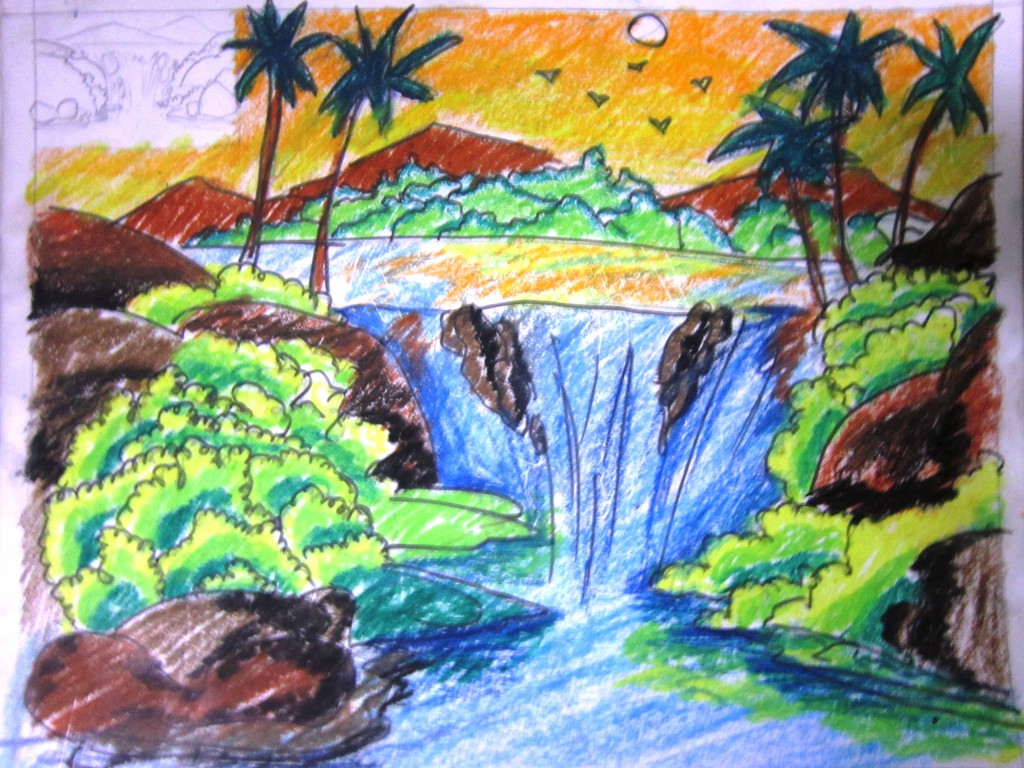A young child colored this vibrant image, likely from a coloring book, depicting a serene waterfall amidst lush greenery. The scene includes various elements such as bushes, palm trees, and distant foliage, adding depth to the landscape. In the foreground, rocks are scattered in the water, showcasing a blend of light brown, dark brown, and blackish-gray hues. The mountainous backdrop enhances the scenic view, while the sky, painted in a mesmerizing yellow-orange gradient, features a central sun and several birds in flight. The trees and bushes exhibit an array of greens—from light to dark—creating a rich tapestry of vegetation. Similarly, the waterfall boasts various shades of blue, contributing to the dynamic composition. Despite the somewhat sloppy coloring indicative of youthful enthusiasm, the image boasts intriguing details and well-coordinated colors, reflecting a charming, creative effort.